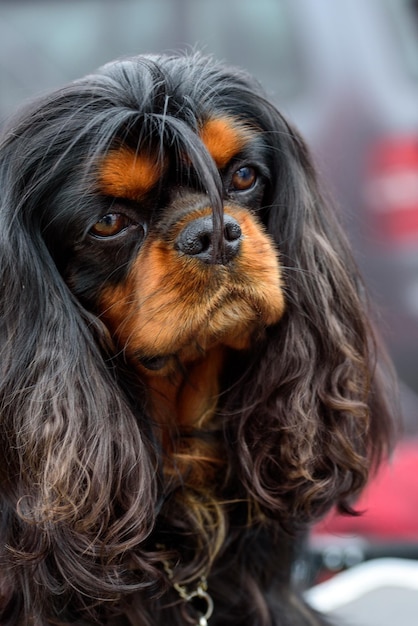This is a detailed portrait photograph of an adult dog with a mysterious breed, showcasing a mix of colors including black, arbonne brown, dark brown, and hints of gray. The dog's face is in sharp focus, highlighting its expressive brown eyes, dark nose, and distinct features such as brown eyebrows and a light brown muzzle. The dog’s ears droop downward, covered in long, furry hair, with a noticeable piece of hair splashed over its nose, adding to its pensive expression. The background is blurred, revealing only subtle hints of red and white hues. Around its neck, the dog sports a chain that resembles a necklace rather than a collar, with a small metal circle for leash attachment. The texture of the dog's fur is captured in fine detail, making for a striking and intimate depiction of the animal.